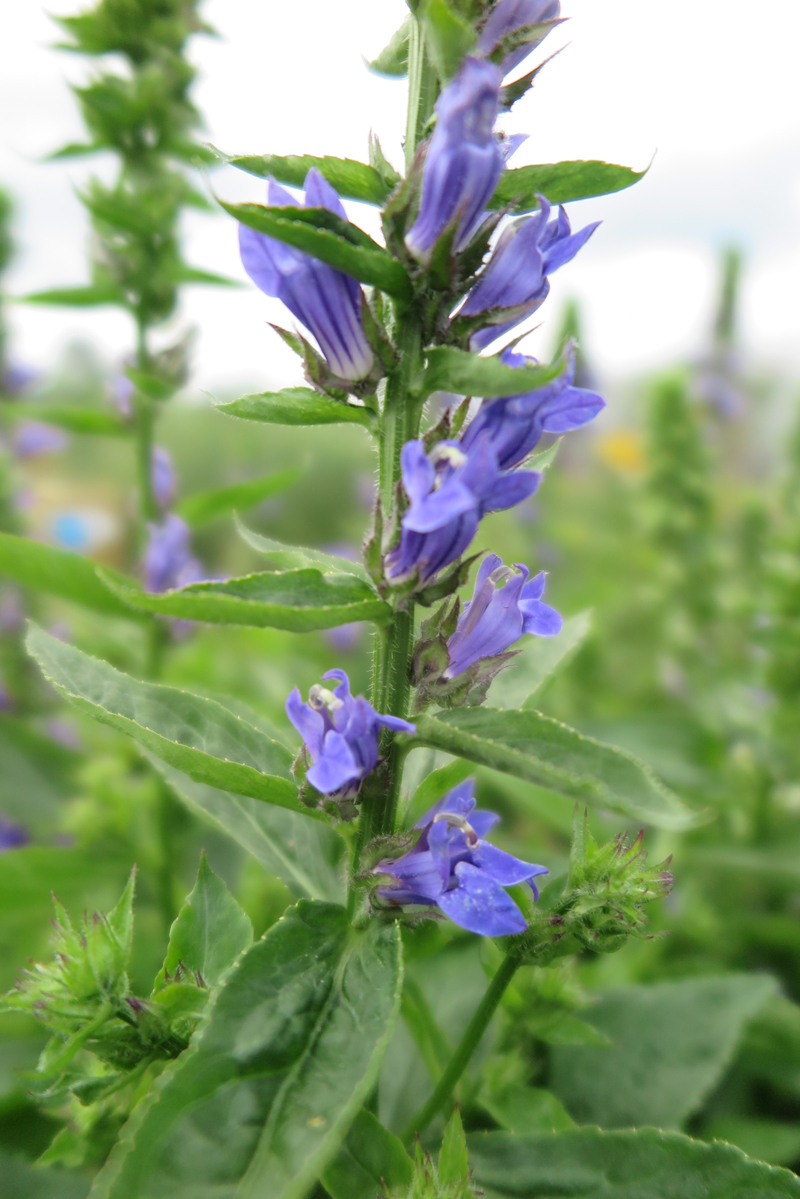The image showcases a close-up of a tall great blue lobelia flower, approximately one foot in height, centrally positioned in the frame. The flower, characterized by its delicate blue bell-shaped petals and dark green stem, is surrounded by buds and deep green, rough-textured leaves that emerge from the base. The background, bathed in soft, hazy light indicative of a bright sunny or overcast summertime day, is artfully blurred, with hints of additional blue lobelia flowers fading into the periphery. This detailed portrayal highlights the newly bloomed freshness of the lobelia, capturing its ephemeral beauty in a serene garden setting likely located in a backyard.